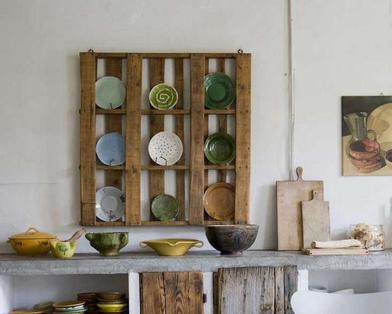This is a photograph of a potentially domestic kitchen or a studio shop, showcasing a beautifully arranged display of handcrafted ceramic items. The main feature is a wooden pallet-like structure mounted on a white wall, which displays nine colorful ceramic plates, arranged in a tic-tac-toe grid. The plates are varied in hues including green, dark green, white, blue, and orange, adding a vibrant touch to the scene. Beneath this wall-mounted display, there is a grey stone counter adorned with an assortment of bowls and handcrafted objects in colors such as orange, green, yellow, grey, gold, brown, and blue. Prominently featured on the counter are a yellow crock and a matching yellow bird figure, alongside green, yellow, and black bowls. To the right of the counter, two cutting boards are propped against the wall. Additionally, a partially visible still life painting, possibly done in acrylic or oil, hangs on the wall near the wooden display, completing the artistic setup.